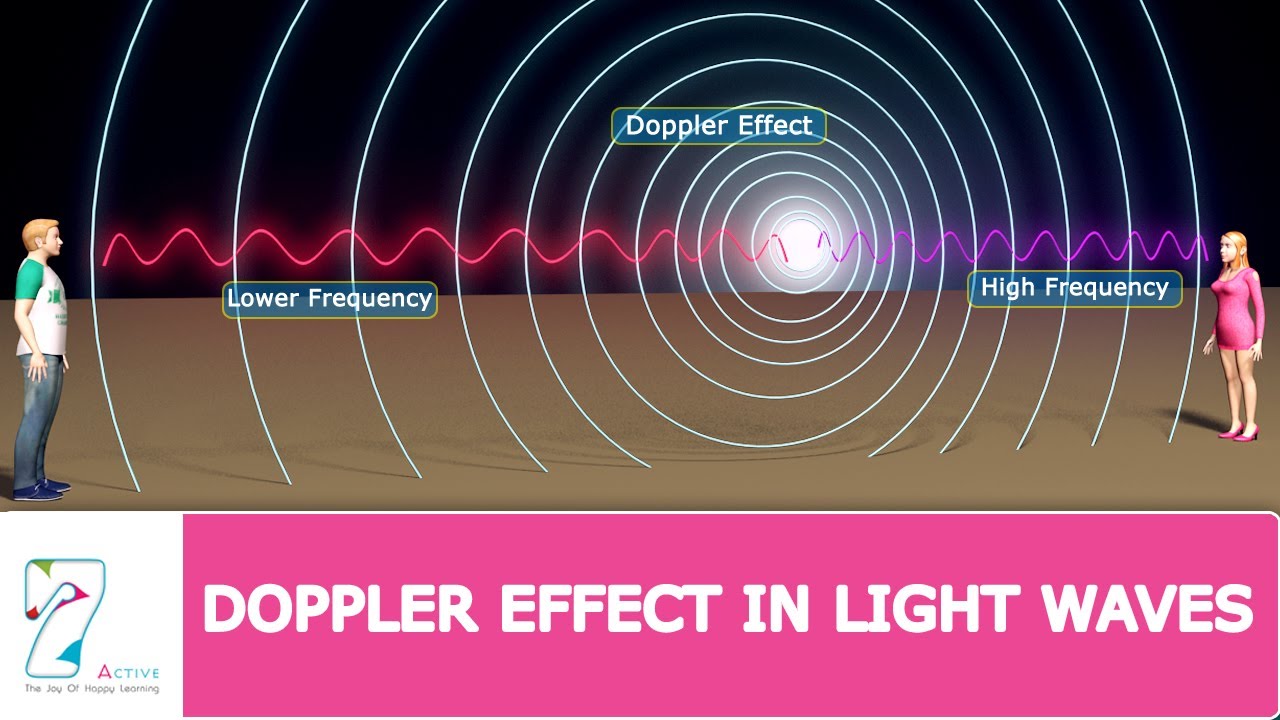The image is a detailed scientific drawing explaining the Doppler effect in light waves, presented by Seven Active, known for promoting joyful learning. At the bottom of the rectangular, panoramic image, there is a pink banner with white lettering that reads "Doppler effect in light waves." In the central part of the image, concentric circles expand outward from a central source, labeled "Doppler effect."

On the left side, a man dressed in blue jeans, a white t-shirt with green sleeves, and blue shoes is depicted. On the opposite side, a woman in a pink dress and high heels with shabby blonde hair faces the man. The visual representation between them illustrates the Doppler effect: the woman on the right perceives high-frequency light waves, depicted with closely spaced purple circles and a squiggled purple line extending towards her. In contrast, the man on the left perceives lower frequency light waves, shown with wider spaced red circles and a red squiggled line.

This detailed illustration effectively demonstrates how light wave frequencies alter depending on the observer's position relative to the source, visually emphasizing the change in frequency through color and spacing of the light waves. The middle features a bright white circle, anchoring the depiction and highlighting the wave's source.